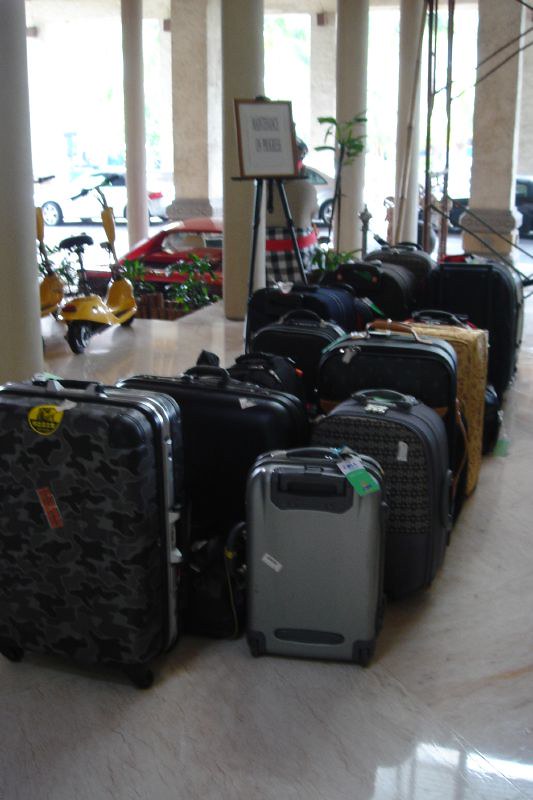The image depicts a somewhat out-of-focus scene outside what appears to be a hotel or convention center, featuring a large assemblage of luggage. Approximately 14 suitcases of varying sizes and colors are prominently positioned side-by-side, mostly upright. They are arranged in neat rows, suggesting an organized setting such as a reception area or lobby entrance. 

The largest suitcase, located at the back, displays a distinctive grey camouflage design. Alongside it is a smaller grey suitcase, surrounded by numerous dark-colored pieces of luggage. There's a notable gold suitcase and a small bag laying on the ground among the upright suitcases. Some of the luggage items bear stickers, including a black and grey camouflage one adorned with yellow and red stickers.

An open area surrounds the luggage, likely the hotel drop-off zone. In the background, large stone pillars and a blurred-out sign on an easel indicate the setting's public nature. To the left of the luggage, two yellow scooters with seats are visible, suggesting off-street parking. At the farthest point, several cars, including a white, blue, and red one, are discernible. Additionally, a figure dressed in a black and white outfit with a red stripe appears in the scene, further contributing to the busy, active atmosphere. The overall impression is one of transit and organization amidst a bustling public space.